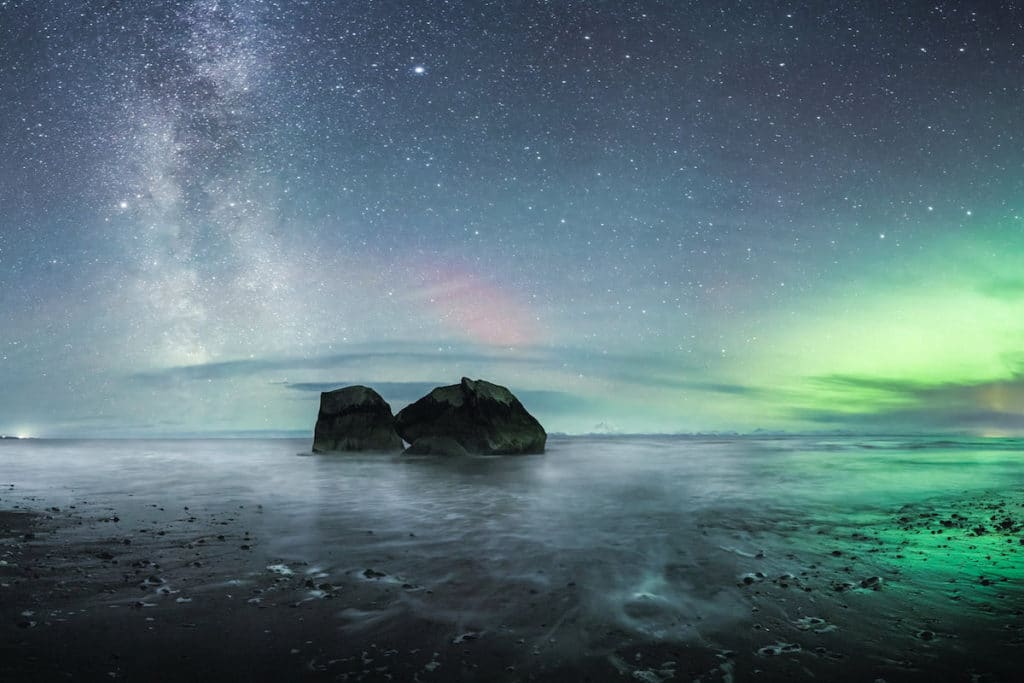This incredibly detailed and enchanting nighttime photograph captures a fantastical scene that blurs the lines between reality and illustration. Dominating the image is a starry sky adorned with white stars and vibrant, hazy swirls of the Northern Lights in green, pink, and a hint of purple, casting an ethereal glow on the entire scene. The awe-inspiring sky reflects its colors on a tranquil body of water that occupies the right-hand corner of the image. Central to the composition are two towering rock formations, resembling large boulders or mountainous structures. The left boulder is rounded, while the right one is wider and disc-shaped. Beneath these formations, the shoreline is visible with scattered pebbles and possibly wet sand, blending seamlessly into the gray, wispy water. At the very bottom of the image, small stones are dotted around, adding texture to the scene. Far across the water to the center left, distant mountains can be discerned, lending depth to the vista. On the far right, faint lights suggest human presence, either from a distant ship or structures on the shore. Overall, the photograph beautifully melds natural elements with celestial phenomena, creating a mesmerizing and almost surreal landscape.